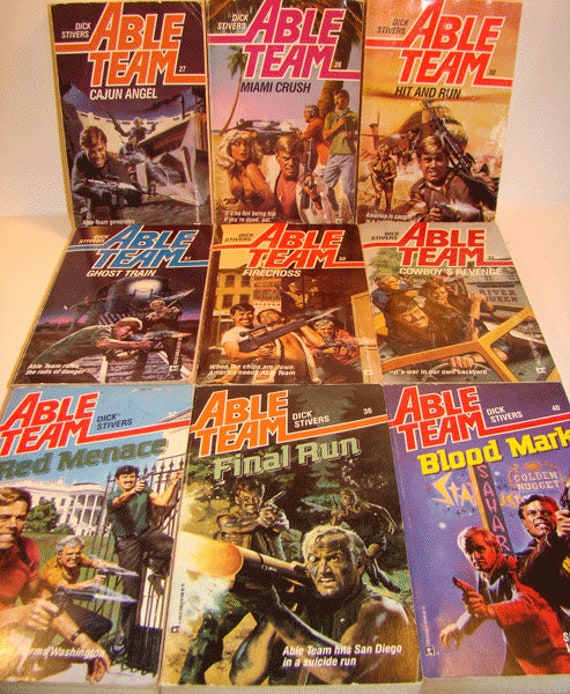This photograph showcases nine comic books from the "Able Team" series by Dick Stivers, meticulously arranged against a stark white background. The composition features six issues laid flat at the bottom and three prominently leaned against a wall in the top third of the frame. Each cover is vividly labeled in either orange, pink, or blue text with titles such as "Cajun Angel," "Miami Crush," "Hit and Run," "Ghost Train," "Firecross," "Cowboy's Revenge," "Red Menace," "Final Run," and "Bloodmark." Central to each cover is a depiction of a short-haired blonde man wielding a gun, set against diverse and dynamic backgrounds that suggest intense action. 

Specific scenarios on the covers include:
- Top left: The primary character with two others against a white building.
- Center top: Two characters leaning against a palm tree with another near the protagonist.
- Top right: The protagonist beside a large helicopter and an additional character.
- Center left: The man and two others around a shiny black object.
- Very center: The protagonist gripping another man by the neck with a third man in the background holding a gun.
- Right: Several characters, including a figure in a boat.
- Bottom left: The scene set in front of the White House with two other men.
- Bottom center: The primary character with a man holding a bazooka and two more characters behind.
- Bottom right: A character illuminated in red with a vertical sign reading "Sahar" behind them.

Overall, the covers suggest a series filled with action and intrigue, each brimming with unique characters and scenarios.